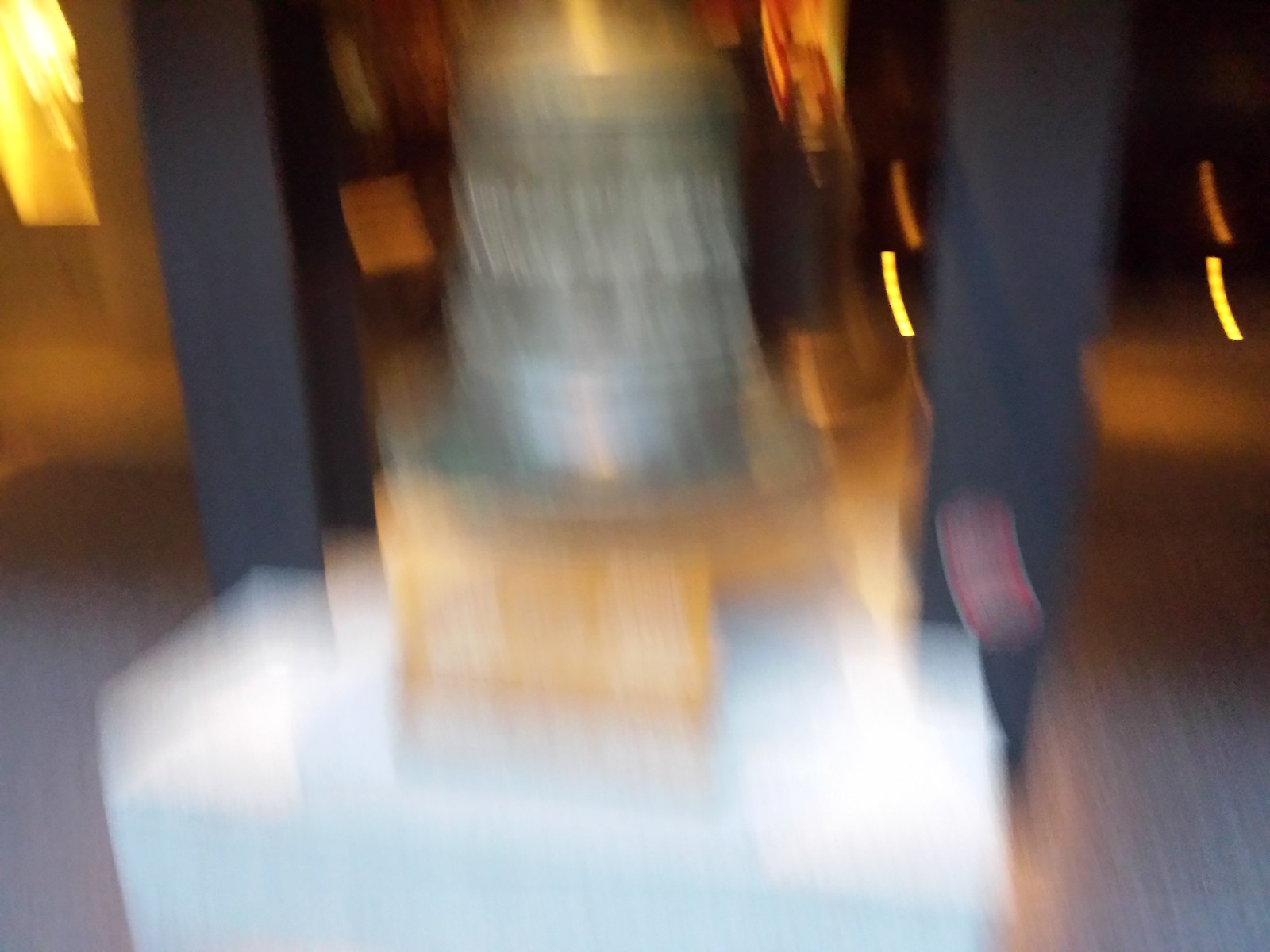This image is a horizontally-oriented, blurry color photograph likely taken indoors in a dimly lit environment, possibly a museum. The central focus is an ornate, historical bell, possibly made of polished bronze or brass, approximately three to four feet tall. The bell is flanked by two vertical black columns and rests on a rectangular white pedestal, which appears to bear an indistinct yellow sign. The background is dark with streaks of yellow lights, suggesting various light sources. The foreground hints at carpeting or a gray floor, further contributing to the impression that this is an indoor setting showcasing historical artifacts. The photograph's extreme blurriness and visible motion blur make it challenging to discern finer details or read any text present.